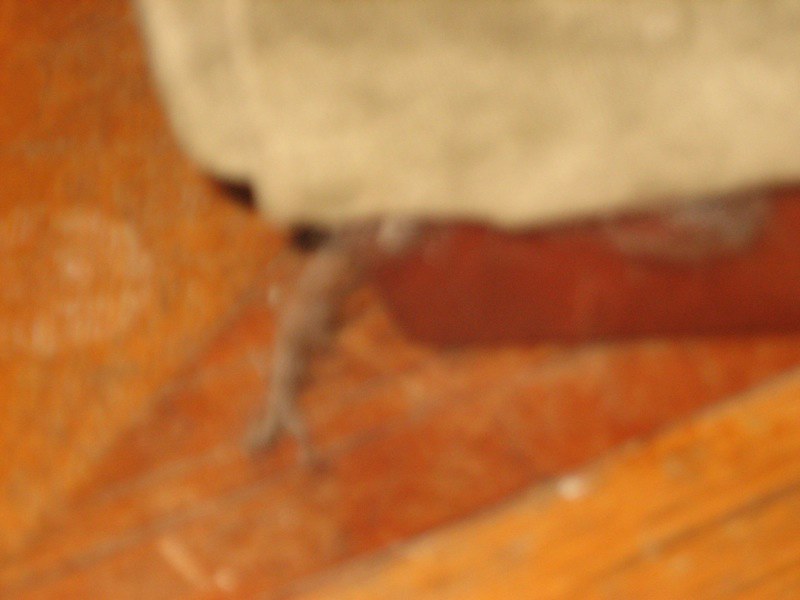This blurry and unfocused image captures a section of a living room floor. The right-hand side of the photo is dominated by what appears to be a brown wooden table, its edge slightly obscured. The table is situated near an orange rug whose vibrant hue closely matches the color of the table, blending the two elements almost indistinguishably. Above the rug, towards the top right corner, there is another piece of fabric that contrasts subtly with the orange rug, suggesting the presence of a cushion or upholstery. Emerging from this fabric is a brown object that bears a resemblance to a branch, extending downwards and touching the floor, adding to the ambiguity and intrigue of the scene. The overall composition is fuzzy and difficult to discern, lending the image an abstract, almost whimsical quality.